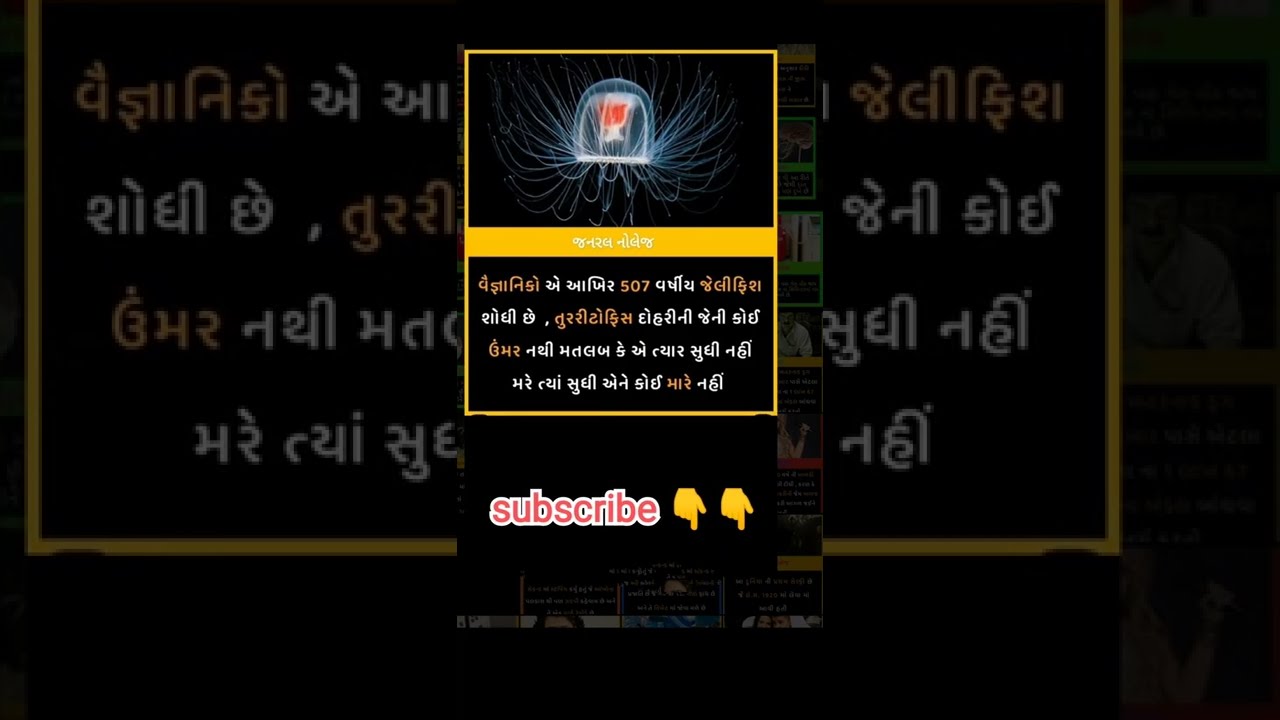The image appears to be a screen grab from a social media video, possibly for TikTok or a YouTube reel. The predominant color scheme features a black background with a prominent yellow border enclosing the main content. At the top, within a rectangular section, there is an image of a ghostly, translucent jellyfish, characterized by its wispy tentacles and a distinct red spot at its center. Surrounding this central image is text in an unfamiliar foreign script, colored in orange and white, which appears on both sides and below the rectangle containing the jellyfish.

Beneath the jellyfish image, there's additional text in the same foreign script. The bottom portion of the image includes a prominent "subscribe" caption in a pinkish hue, accompanied by two yellow hand icons on the right, with their pointer fingers and thumbs directed downward, indicating a call to action. Small, indistinct pictures are located to the right and below the main yellow-bordered rectangle, but they are not clearly visible. The overall layout suggests the image functions as an advertisement or pop-up designed to engage viewers and encourage them to subscribe.